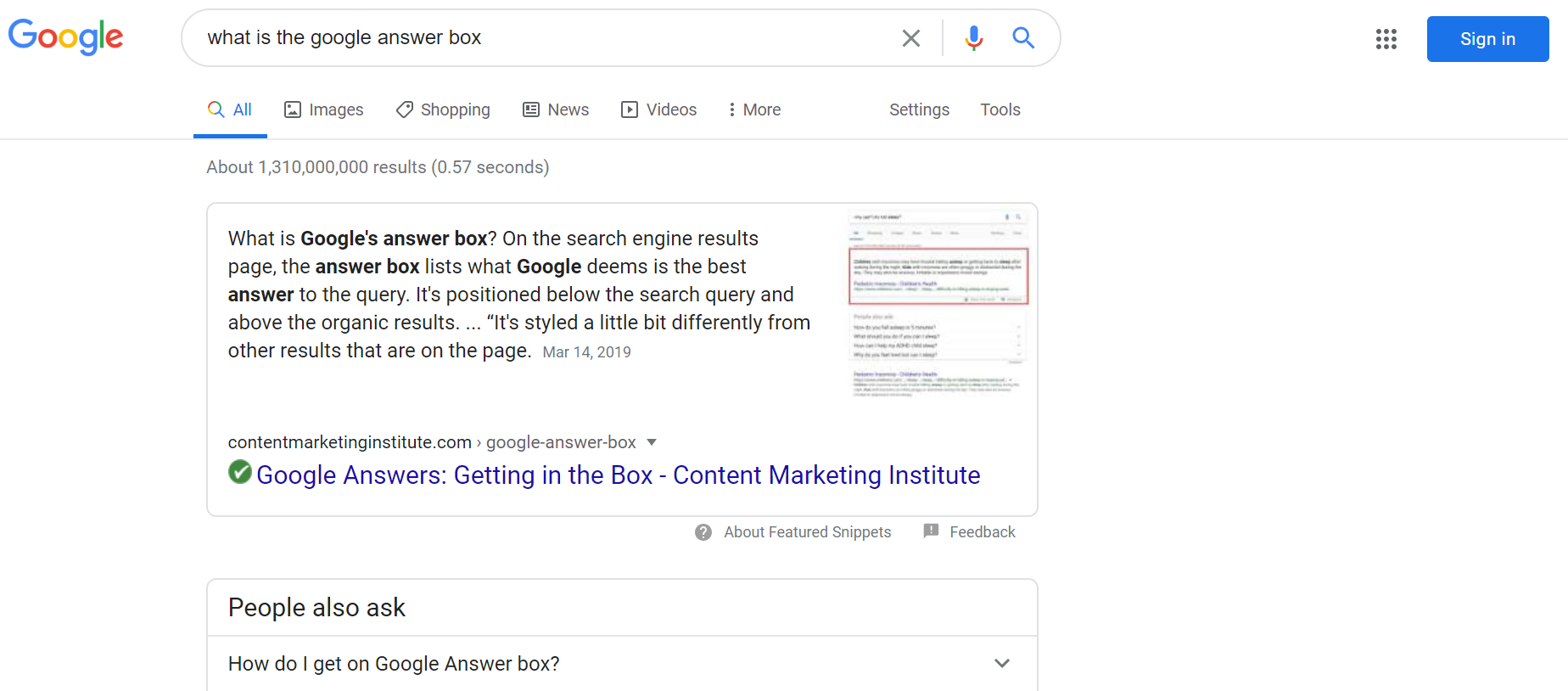A computer screen displays a Google search results page under the query "What is Google's answer box?" At the top of the screen, a microphone icon, magnifying glass, 9-dot grid, and "Sign in" option are visible beside the navigation tabs for all images, shopping, news, videos, more, settings, and tools. 

Prominently featured below the search bar, Google's answer box highlights the most pertinent response to the user query, positioned above other traditional search results. The box content suggests a concise definition, stating that Google's answer box is designed to provide the best possible answer to a query. 

The screen captures the results from Content Marketing Institute, displaying links about the Google answer box, how to get your content featured, and related feedback options. Visually, the background is white with clear dividers between different sections and snippets of text. The search results claim to be from approximately 1.31 billion entries found in about 0.5 seconds, showcasing Google's efficiency and vast information coverage.

Additionally, the image features related queries such as "how do I get on Google's answer box," illustrating different kinds of lines and dividers in a white background layout. The result set emphasizes the structured and easily navigable design of Google's interface to facilitate quick access to sought-after information.